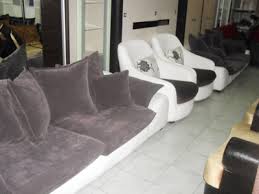The image is a small, low-resolution, color photograph depicting a room filled with a variety of couches and individual armchairs, suggesting it might be a furniture store or warehouse. The furniture is arranged in rows, with one stretching from the front left corner to the back right corner, and another partial row in the foreground. The floor is a reflective, high-shine, gloss ceramic tile with a pattern of squares and darker parallel lines. 

In the foreground, there is what seems to be a two-seater couch with wine-colored bottom cushions and matching back cushions, set against a white leather frame. To its right, two individual armchairs also have white leather surrounds but feature dark seat cushions. Further along, the next couch has grey cushions that appear very soft, again with a white base. Adjacent to these are two white armchairs and another similar couch with grey cushions and a white frame. Toward the back right of the image is a white sofa with black seat cushions, and across from it, on the opposite side, are wooden chairs with yellow or gold seat cushions. The background includes a white wall with several brown doors or windows behind the primary line of furniture. The detailed arrangement and diverse styles of the furniture in a well-lit, glossy-tiled room enhance the likelihood that this is a commercial setting, possibly a waiting area or a furniture showroom.